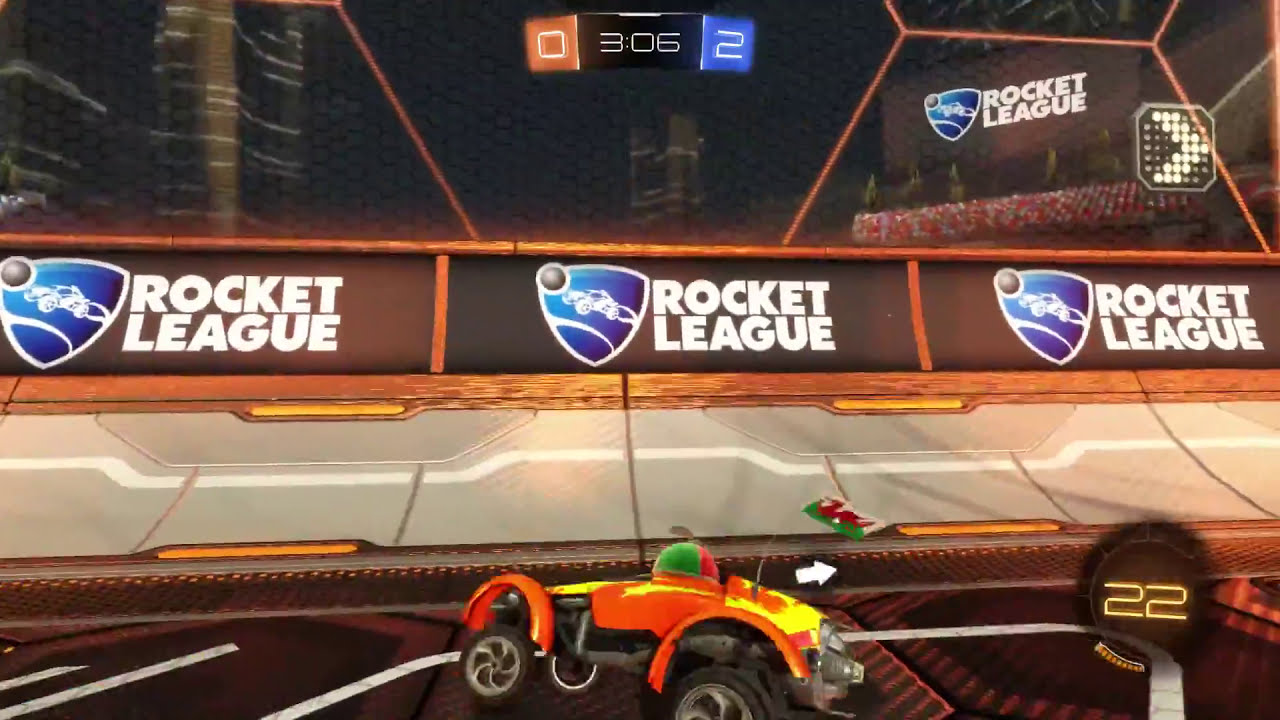The image is a detailed screenshot from the video game Rocket League, showcasing a competitive match. The scene captures an older-style racing arena with vibrant, somewhat dated graphics. Dominating the lower part of the frame is a distinct red and yellow retro cigar-shaped racing car situated on the track. The surrounding stadium, colored in orange and gray tones, features a cage wall with the "Rocket League" logo prominently displayed in large white block letters three times, left, center, and right, accompanied by a blue shield symbol. The top section of the image includes a black strip displaying the game timer, indicating three minutes and six seconds remaining, with the score at zero for orange and two for blue. Additional details include a smaller timer showing 22 seconds at the bottom right and a notable arrow indicator for the ball pointing right. The car is adorned with a hat, adding to the lively, colorful atmosphere of the game.